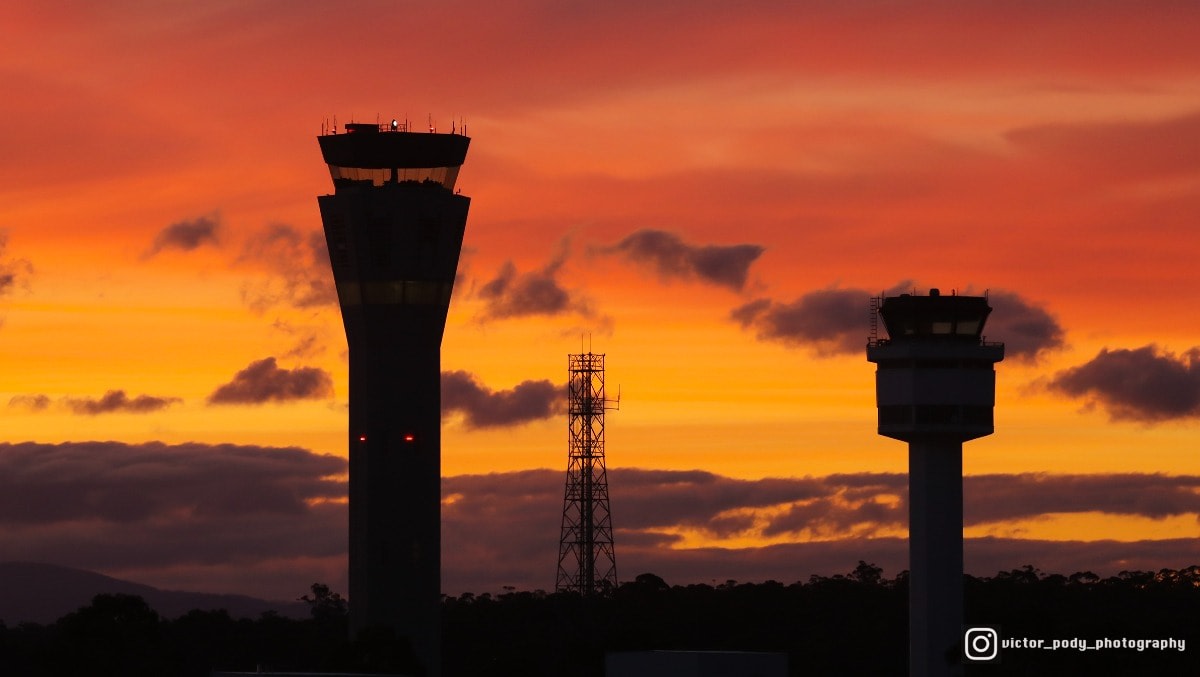The outdoor photograph, taken at dusk, captures a dramatic scene with deep contrasts and vivid colors. In the center left, a prominent air traffic control tower stands, silhouetted against the vibrant sky, with only a few side lights faintly illuminating its structure. The tower's windows reveal patches of the sky beyond. On the far right, a smaller air traffic control tower mirrors its larger counterpart, both enveloped in shadow. Between them, in the distant background, a radio tower rises against a landscape of silhouetted trees, adding depth to the composition.

The sky itself is a breathtaking gradient, starting with dark grey clouds near the horizon, transitioning to a brilliant orange that intensifies to red and darkens as it ascends. This colorful display clearly marks the time of sunset. In the bottom right corner, the photo features an Instagram logo and the white text "Victor Poggi Photography," indicating the source of this evocative image.